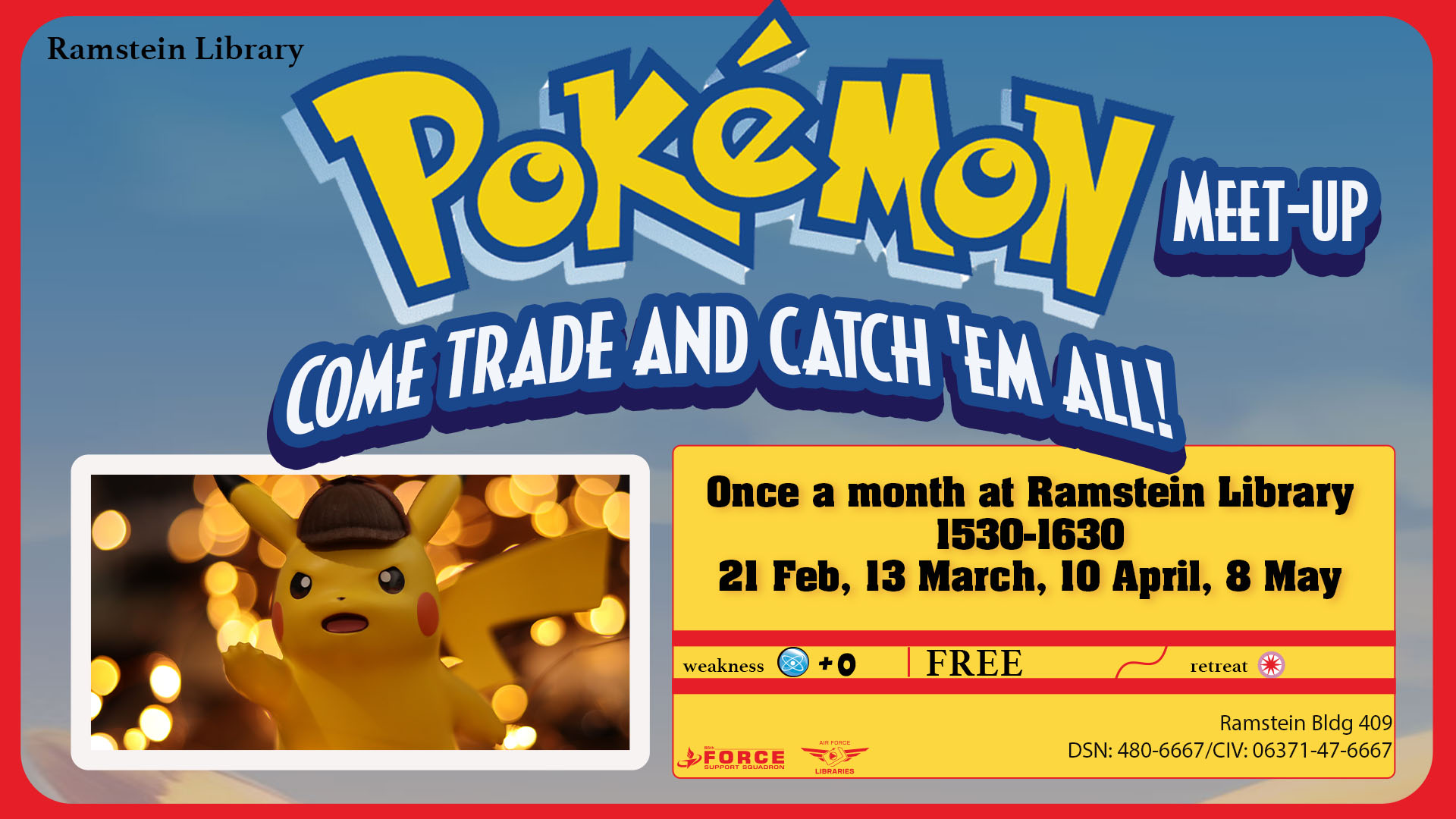Here's the cleaned up and detailed caption for the image:

---

The poster advertises a Pokémon Meetup event at Ramstein Library. The design features a vibrant red rectangular background, overlaid with a rounded-corner blue image that almost fully covers the red backdrop. This blue image resembles a sky scene with brown and yellow clouds or mountains at the bottom corners. In the top left, "Ramstein Library" is written in black text. At the center top, the iconic Pokémon logo stands out with its yellow lettering, blue highlights, and a light blue to white gradient shadow. To the right of the logo, “Meetup” is written in bold white text with a blue outline and dark blue shadow. Directly below, the phrase “Come Trade and Catch 'Em All” follows in a similar typography style.

Beneath these headings, the poster includes two main visual elements. On the bottom left, there is an image of a Pikachu figurine with a black cap and an intense expression, set against a background of blurred light bokeh circles. On the bottom right, a ticket-like object with a yellow background and thin red outline provides event details in black text, reading: "Once a month at Ramstein Library, 15:30 to 16:30, 21 February, 13 March, 10 April, 8 May."

---

This caption offers a detailed description, capturing both the visual and textual elements of the poster.